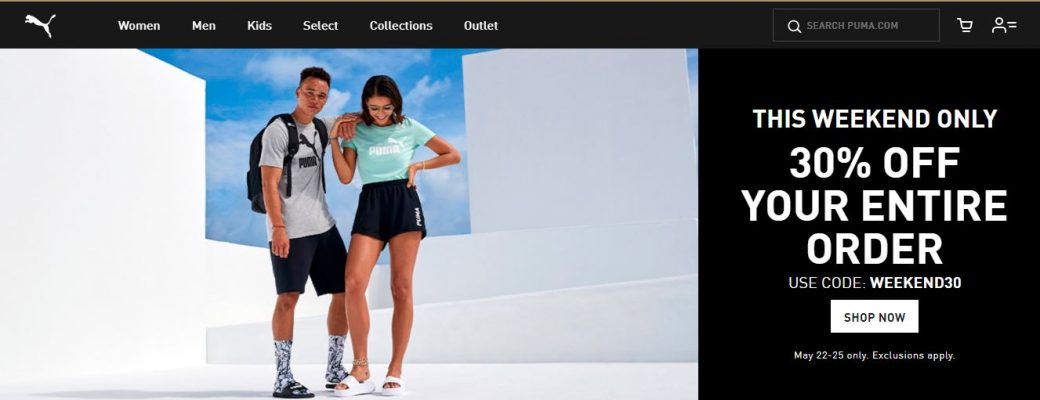The image features the homepage of the Puma website. In the top left corner, the iconic white Puma logo - a leaping wildcat - is set against a black background. The website's main navigation menu is displayed at the top, featuring categories such as Women, Men, Kids, Select, Collections, and Outlet. To the right of the menu, there's a search bar with the placeholder text "searchpuma.com," accompanied by a white magnifying glass icon. Further to the right, there are icons representing a shopping cart and a user profile.

Directly below the navigation bar, bold white text reads: "THIS WEEKEND ONLY, 30% OFF YOUR ENTIRE ORDER. USE CODE: WEEKEND30." A white "Shop Now" button with black text is prominently displayed beneath this message, and an additional note states, "May 22nd to 25th only, exclusions apply."

On the left side of the image is a photo featuring a man and a woman. The man is wearing a black backpack, black shorts, and black and white socks. His hand rests on the shoulder of the woman, who is dressed in a green shirt, black shorts, and white sandals. Both individuals are sporting Puma-branded apparel. They are positioned in a bright, white setting with a backdrop of blue sky and fluffy clouds.